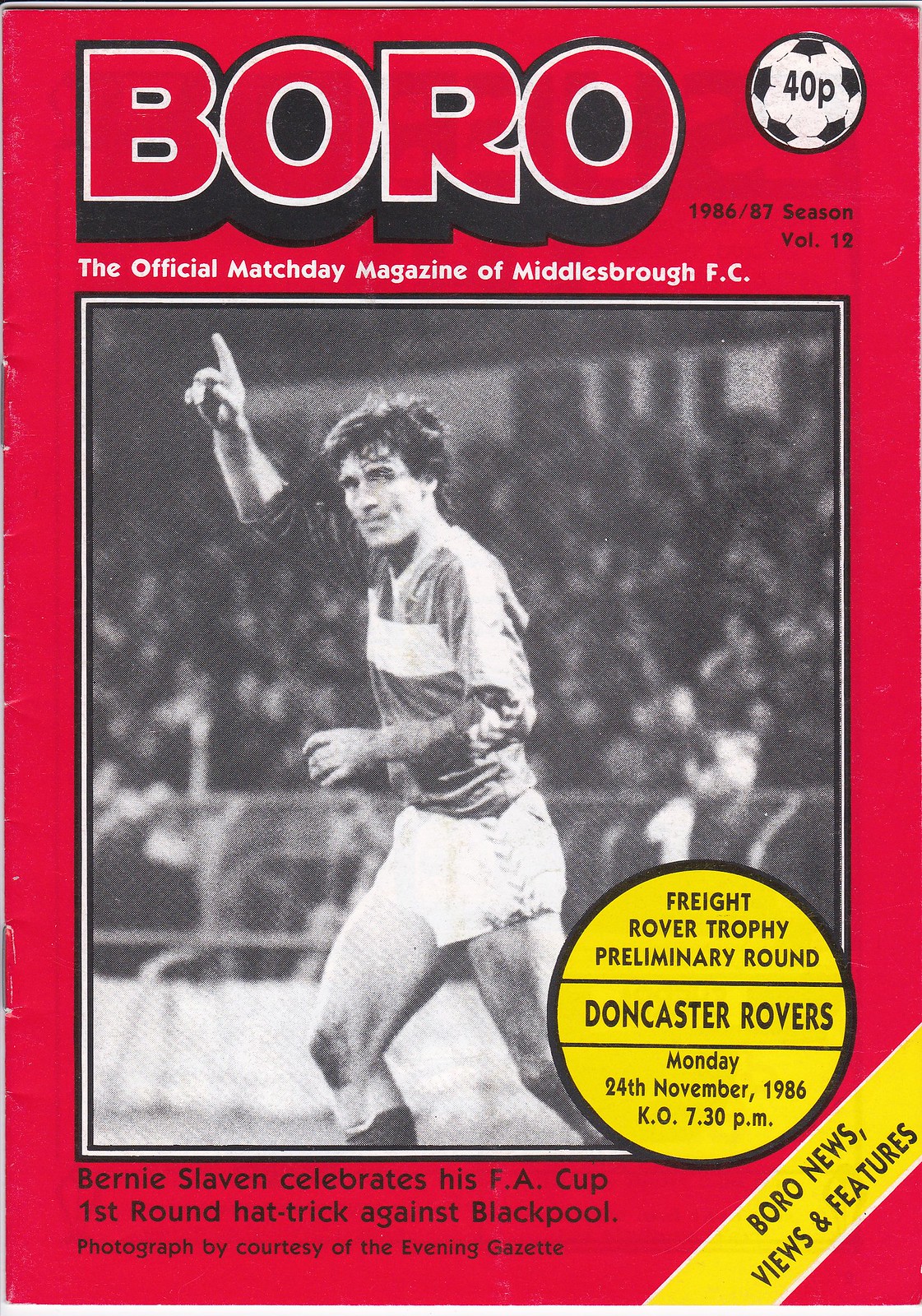This is the cover of the official Match Day program for Middlesbrough FC, from the 1986-87 season, Volume 12. The background is entirely red. At the top, large text reads "BORO" in all capital letters, styled in red with a white border and a solid black drop shadow. In the top right corner, there's a small soccer ball icon with "40P" written inside, indicating the price. Just below "BORO," small white text states "The Official Match Day Magazine of Middlesbrough FC."

The centerpiece of the cover is a large black and white photograph of a soccer player pointing upwards with his right arm, making the number one symbol. He has short brown hair and is dressed in a jersey featuring a white stripe through the middle, paired with light-colored shorts. Overlapping the bottom right of this photo is a yellow badge that reads "Freight Rover Trophy Preliminary Round, Doncaster Rovers, Monday, 24th November 1986, Kickoff 7.30 p.m." A caption beneath the photograph, in black text, reads "Bernie Slavin celebrates his FA Cup first round hat trick against Blackpool, photographed by courtesy of the Evening Gazette."